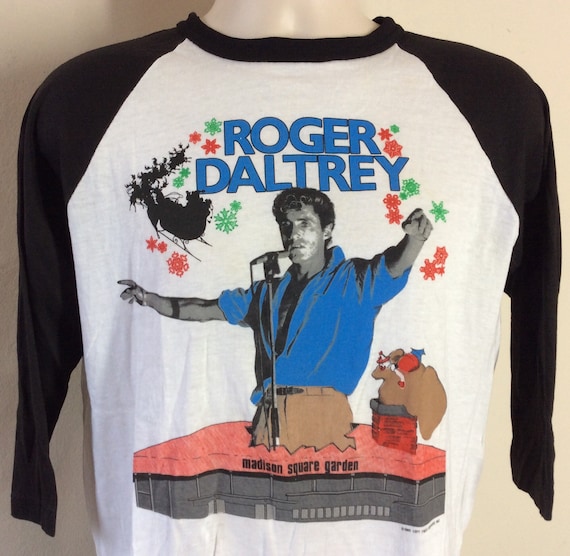A stylish baseball-style t-shirt is exhibited in this image. The design features contrasting black sleeves and a white body. Central to the design is an artistic depiction of Roger Daltrey, prominently showcased standing atop a drawing of Madison Square Garden. Surrounding this central image, whimsical holiday details abound: a black silhouette of Santa in his sleigh pulled by reindeer, nearing a chimney from which a sack of toys seems to emerge. A festive flair is added with red and green snowflakes scattered across the shirt. Roger Daltrey is illustrated wearing a blue shirt paired with tan trousers. The shirt is displayed on a mannequin against a cream backdrop, highlighting its unique and celebratory design.